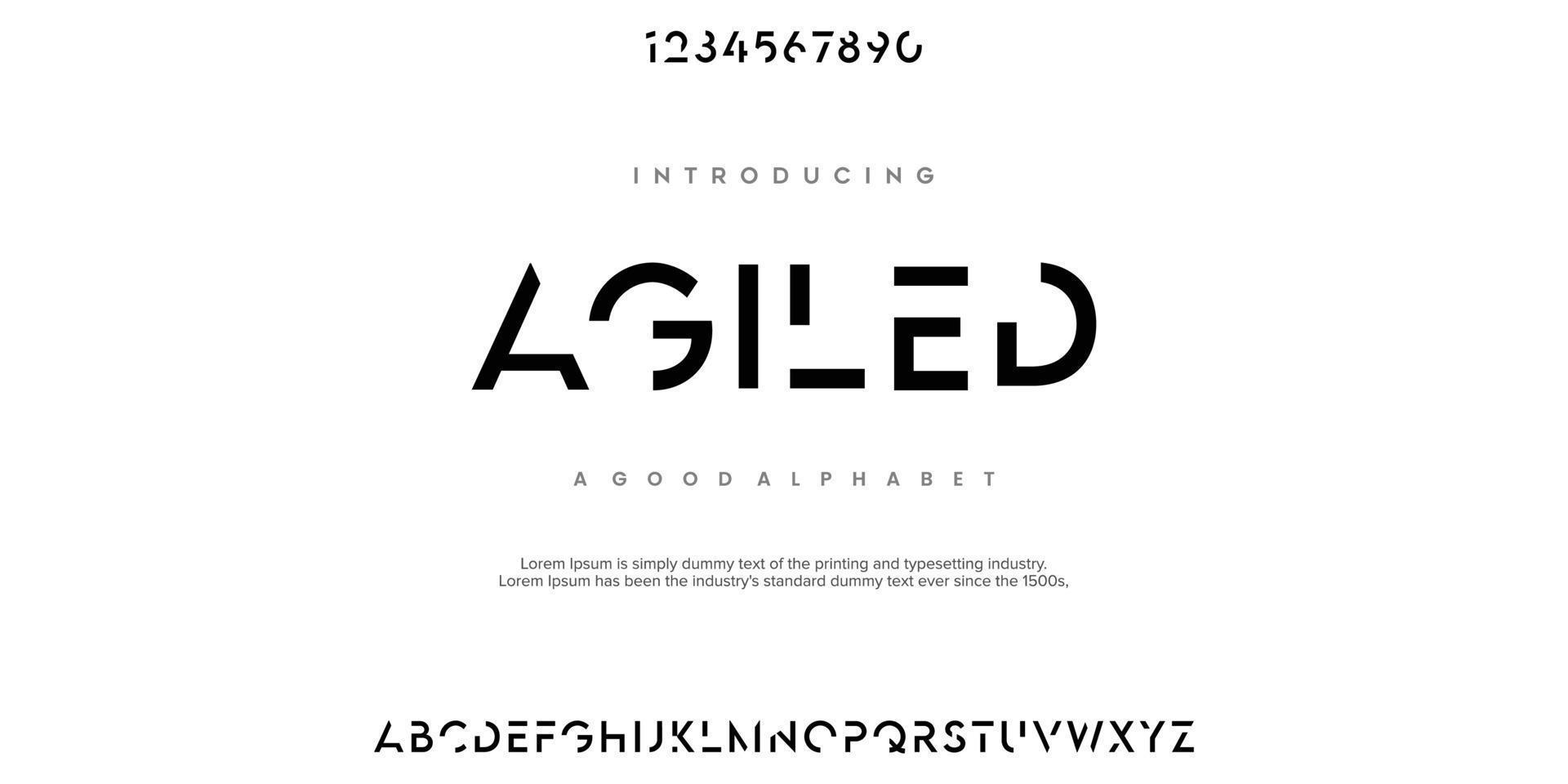The image depicts a white background with a series of black text and numbers, all featuring a unique font with missing pieces. At the top, it displays the numbers 1 through 9, followed by 0, each number noticeably having chunks missing but still recognizable. Below the numbers, the text reads "INTRODUCING A-G-I-L-E-D," where each letter also has portions missing. Further down, it states "A GOOD ALPHABET," followed by a block of placeholder text starting with "Lorem Ipsum is simply dummy text of the printing and typesetting industry. Lorem Ipsum has been the industry's standard dummy text ever since the 1500s." Finally, at the bottom of the image, the complete alphabet is presented in the same fragmented font style, from A to Z, with portions of each letter missing.